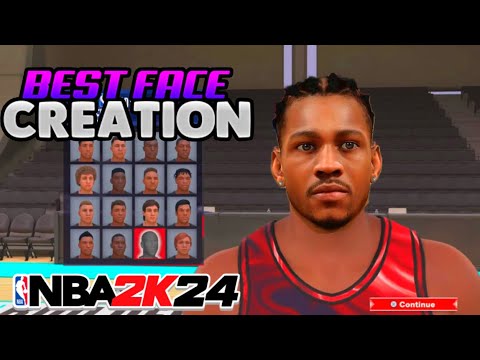Screenshot from the video game NBA 2K24 depicting a computer-generated image of a famous basketball player. The game's title, "NBA 2K24," is prominently displayed, with "2K" in red and "NBA 24" in black with a white outline. On the left side of the image, there's a yearbook-style chart featuring multiple profile pictures of players, labeled "Best Face Creation." The word "Best" is in purple, while "Face Creation" is in gray. In the lower part of the chart, the third picture from the fourth row stands out with a red background and a silhouette of a person's head, whereas the rest of the portraits display distinct human facial features. The player on the right side of the image has cornrows, dark skin, and is wearing a red jersey, indicating an African-American character. Additionally, a red "Continue" button is located at the bottom right corner. The overall background resembles a set of bleachers, adding to the sports game atmosphere.